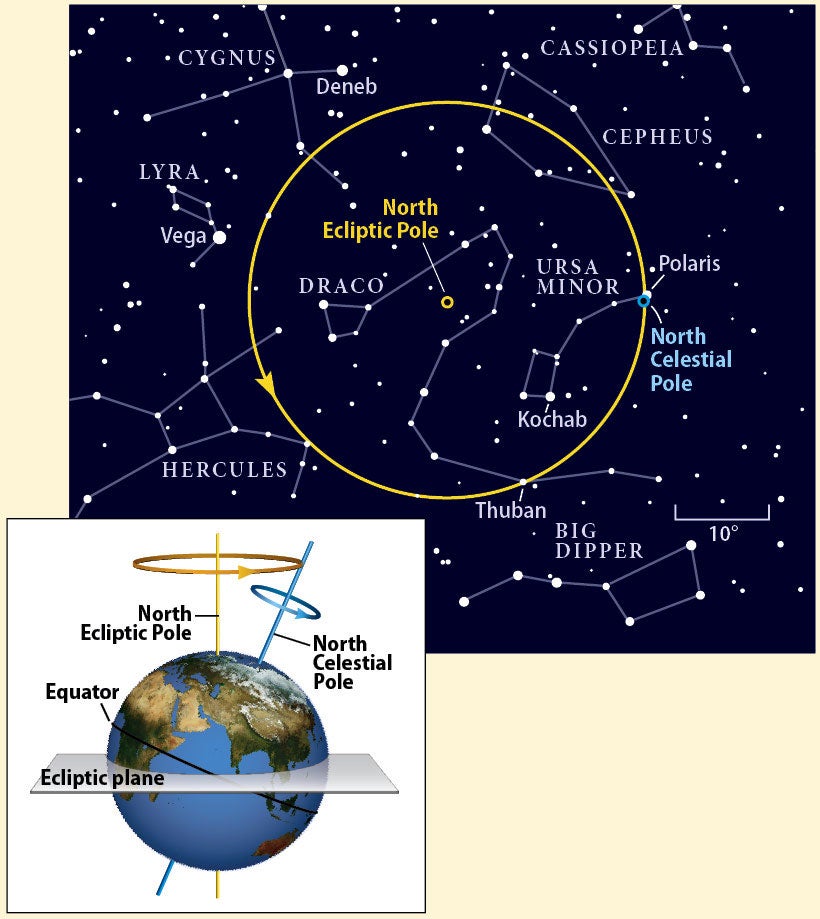The image can be described as an intricately detailed celestial map, predominantly showcasing a dark blue background filled with numerous white star symbols and constellation lines. At the center of the larger central section, there is a prominent yellow circled outline, denoting the North Ecliptic Pole, surrounded by various constellations such as Cygnus, Deneb, Cassiopeia, Cepheus, Ursa Minor, Polaris, Hercules, Vega, Lyra, Big Dipper, and Thuban. These constellations are connected by white lines, adding structure to the starry map. 

Below, specifically at the bottom left corner, the image transitions to a smaller graphic illustrating the Earth. This secondary image highlights the African and Asian continents, marked with significant celestial labels such as the North Celestial Pole, the North Ecliptic Pole, the Equator, and the Ecliptic Plane. The background of this Earth graphic is white, contrasting with the celestial map above, while the Earth itself is depicted in its natural colors. Overall, the image appears to be an educational diagram, possibly from a poster, book, or webpage, meant to convey detailed astronomical information.